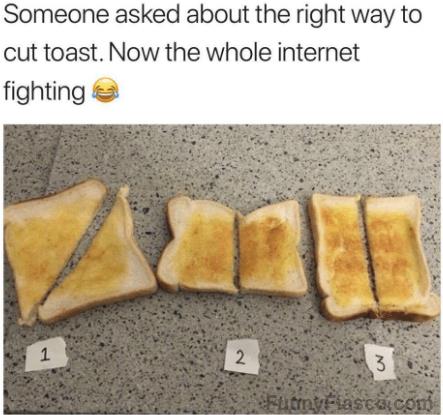The image shows a social media post, featuring a granite countertop with three pieces of white bread toast laid out horizontally. Above the toast is a caption: "Someone asked about the right way to cut toast. Now the whole internet is fighting," accompanied by a laughing-crying emoji. Each piece of toast is evenly spaced and labeled with numbers 1, 2, and 3. Toast number 1 is cut diagonally into two triangular halves. Toast number 2 is sliced vertically into two rectangular halves. Toast number 3 is divided horizontally, creating two long, narrow rectangles. Each slice has visible butter and cinnamon, enhancing their textured appearance. A watermark is present at the bottom of the image.